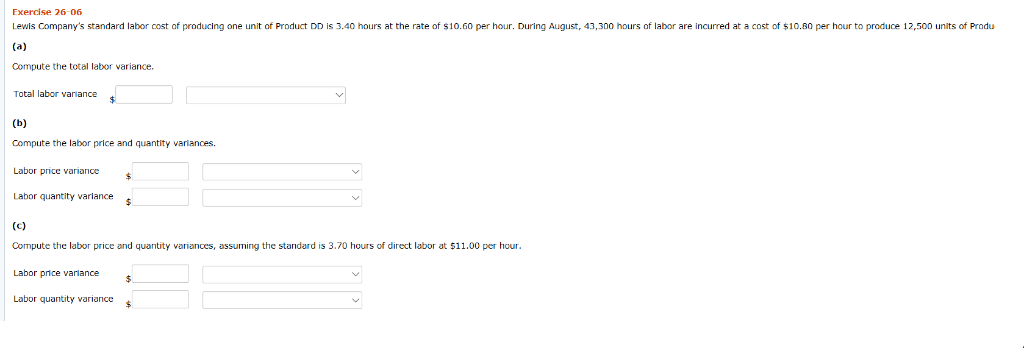The image depicts an online college assignment focused on standard labor cost calculations. The specific problem is labeled "Exercise 26-06: Lewis Company." It involves determining the standard labor cost of producing one unit of product "DD," which is specified as requiring a certain number of hours at a rate of $10,000 per hour. During August, a labor expenditure of 43,300 hours at a cost rate of $10,080 per hour was recorded to produce 12,500 units.

The assignment is divided into three parts:

1. **Part A: Calculate the Total Labor Variance**
   - A prompt asks for the "Total Labor Variance" with a dollar sign and a box for the answer.

2. **Part B: Compute the Labor Price and Quantity Variances**
   - This section requires the labor price variance and labor quantity variance to be calculated. Each variance has a corresponding dollar sign and box for the answer, with dropdown menus or options for selection.

3. **Part C: Compute the Labor Price and Quantity Variances Based on Standard Assumptions**
   - Using a standard of 3.70 hours of direct labor at $11 per hour, the assignment asks for recalculation of the labor price variance and labor quantity variance. Similar to Part B, each calculation has a dollar sign, answer box, and additional options for input.

This detailed description helps to capture the essence and requirements of the online assignment, providing clear guidance on the tasks at hand.